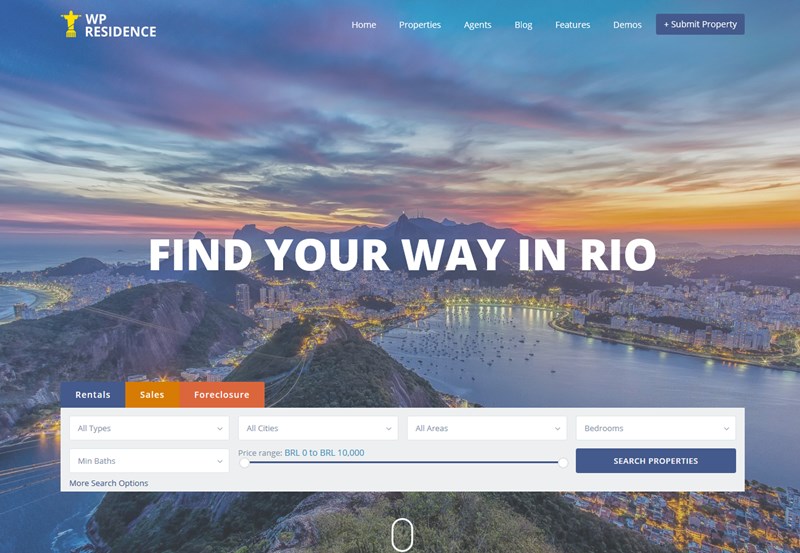The image depicts a web page from the WP Residence website, designed for property listings. Prominently displayed at the top right, in white text, it reads "WP Residence" accompanied by a gold statue logo. The navigation menu features links labeled as "Home," "Properties," "Agents," "Blog," "Features," "Demos," and a "Submit Property" button in blue.

Dominating the top of the page in large white font is the phrase "Find Your Way in Rio," set against an aerial view of a cityscape at dusk. The background captures a vibrant, colorful sky that transitions from shades of orange to blues and purples as the sun sets over the mountains. The mountains themselves are a mix of green and brown hues, and a serene waterway snakes through the city, reflecting the myriad lights from nearby buildings. Boats float peacefully on the water, enhancing the tranquil, scenic beauty of the evening.

The cityscape reveals an array of white buildings spread across the landscape, indicative of a bustling and vibrant urban area. At the bottom of the page, there is a search bar with options for "Rentals," which has a blue background, "Sales" marked in orange, and "Foreclosures" highlighted in red. Additionally, there are several drop-down menus for filtering search results by property type, city, area, the number of bedrooms, and bathrooms. The search functionality is completed with a blue "Search Properties" bar.